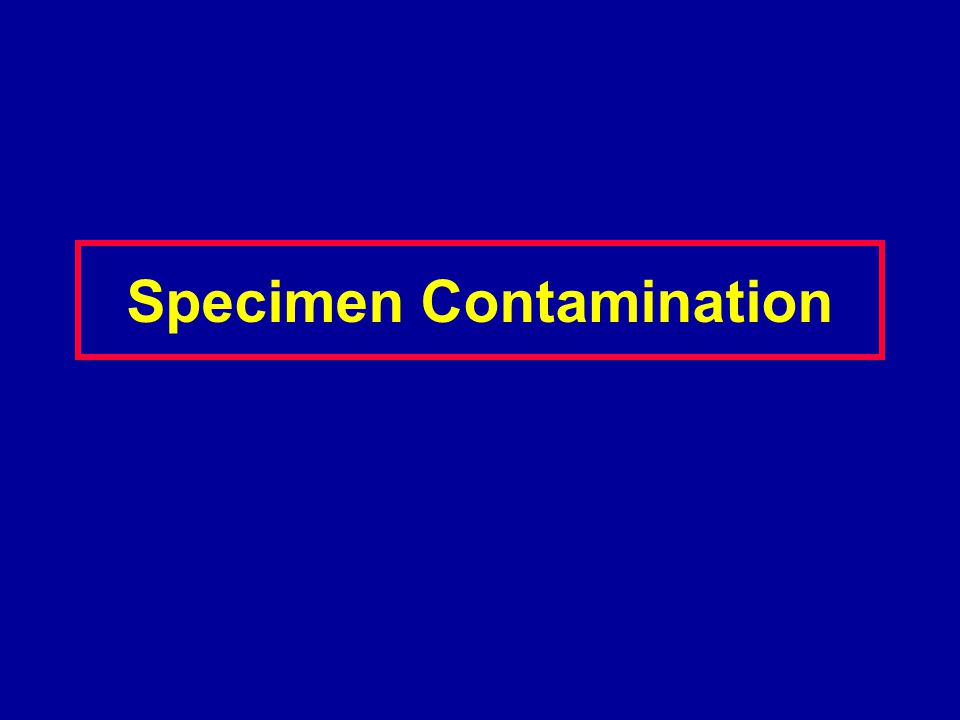The image features a dark blue background with a centrally positioned, almost square-shaped slide. Slightly above the center of this dark blue backdrop, there is a prominent red rectangle that stretches nearly the entire width of the slide. Inside this red rectangle, there's the text "Specimen Contamination" written in yellow, capitalized letters. The yellow text is framed against the blue background, encased within the red border. The simple yet striking color palette consists of dark blue, red, and yellow. The image likely serves as a presentation slide, possibly for educational or informational purposes, and the text appears to be in a standard font like Arial.